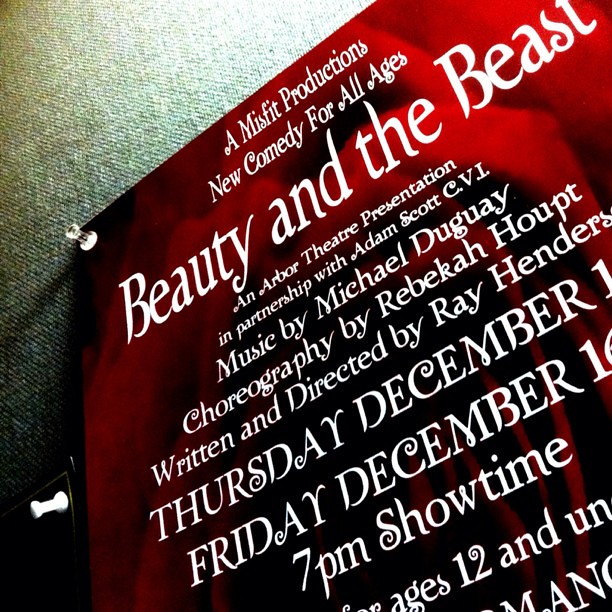The image depicts a color photograph of the upper portion of a red poster promoting a theater performance. The poster is pinned to a cloth bulletin board with a transparent pushpin in the upper left corner. Adjacent to it, the corner of another black poster is held in place by a white pushpin. The central design of the poster features a large, close-up image of a rose, providing a striking red background. 

The white text on the poster reads: "A Misfit Productions new comedy for all ages, Beauty and the Beast." It continues with details: "An Arbor Theatre presentation in partnership with Adam Scott CVI, music by Michael Duguay, choreography by Rebecca Haupt, written and directed by Ray Henderson." 

The image cuts off the lower part of the poster, but it partially reveals showtimes: "Thursday December," and "Friday December 16, 7 p.m. Showtime." There is an indication that the performance is suitable for ages 12 and under, though this information is incomplete due to the angle of the photograph.